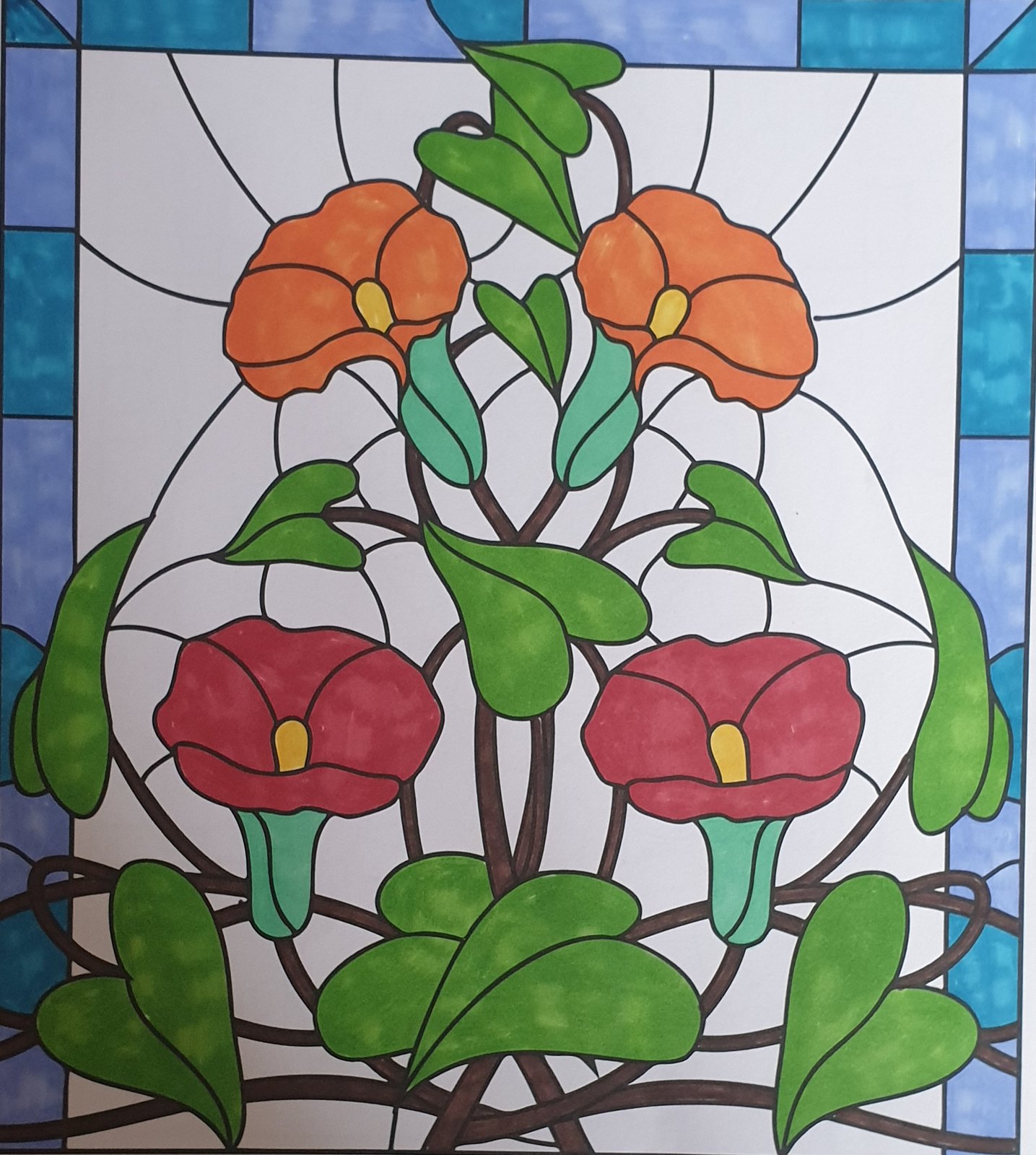This image showcases an artist's imaginative concept for a stained glass window. The design intricately details the components and aesthetic of a stained glass piece. The perimeter of the window features angular glass fragments in shades of aqua blue and gray, bordered by lead strips that underscore the typical stained glass framework. 

The center of the design seamlessly integrates additional lead angles, which gradually give way to a vibrant floral arrangement. Bright orange flowers bloom amidst lush green leaves and darker, earth-toned stems, which curl and weave harmoniously among the leaded lines. The background of the central section is rendered in white, enhancing the vivid colors of the flowers and foliage.

Although this is not a photograph of an actual stained glass window, it vividly captures the essence and elegance of such a piece, blending creative inspiration with detailed design elements. The artist's concept meticulously blends the structured architecture of stained glass with the organic beauty of nature, resulting in a visually captivating and richly detailed composition.